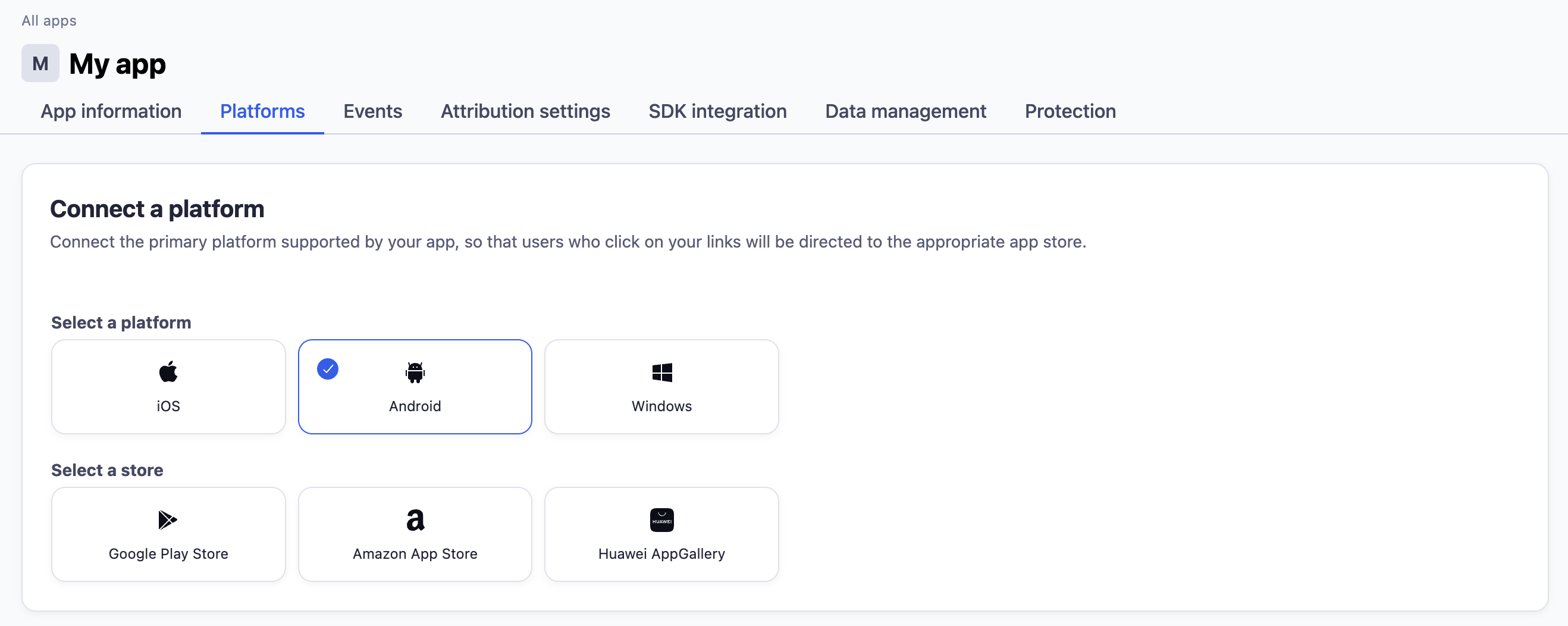The screenshot depicts an app developer tool interface in light mode, characterized by a light grey border and a white main screen with black text. The top left corner features the title "My App" prominently, accompanied by a grey square with a capital "M" in it. Above this, "All Apps" is displayed, indicating that the current view pertains to "My App."

A series of menu options are listed horizontally at the top, including App Information, Platforms, Events, Attribution Settings, SDK Integration, Data Management, and Protection. The Platforms tab is currently selected, highlighted in blue with an underline.

The main content section under Platforms is titled "Connect to Platform," guiding the user to connect their app to a primary platform. This setup ensures users who click on links are directed to the appropriate app store. Below this title are two dropdown menus: "Select a Platform" and "Select a Store."

In the "Select a Platform" dropdown, options include iOS (indicated by the Apple logo), Android (represented by the Android mascot), and Windows (denoted by the Windows symbol). The Android option is currently selected.

Under "Select a Store," the Android-specific options are displayed: Google Play Store (with its arrow icon), Amazon App Store (marked by a capital "A"), and Huawei App Gallery. This section allows configuration of the app's presence in these respective stores.